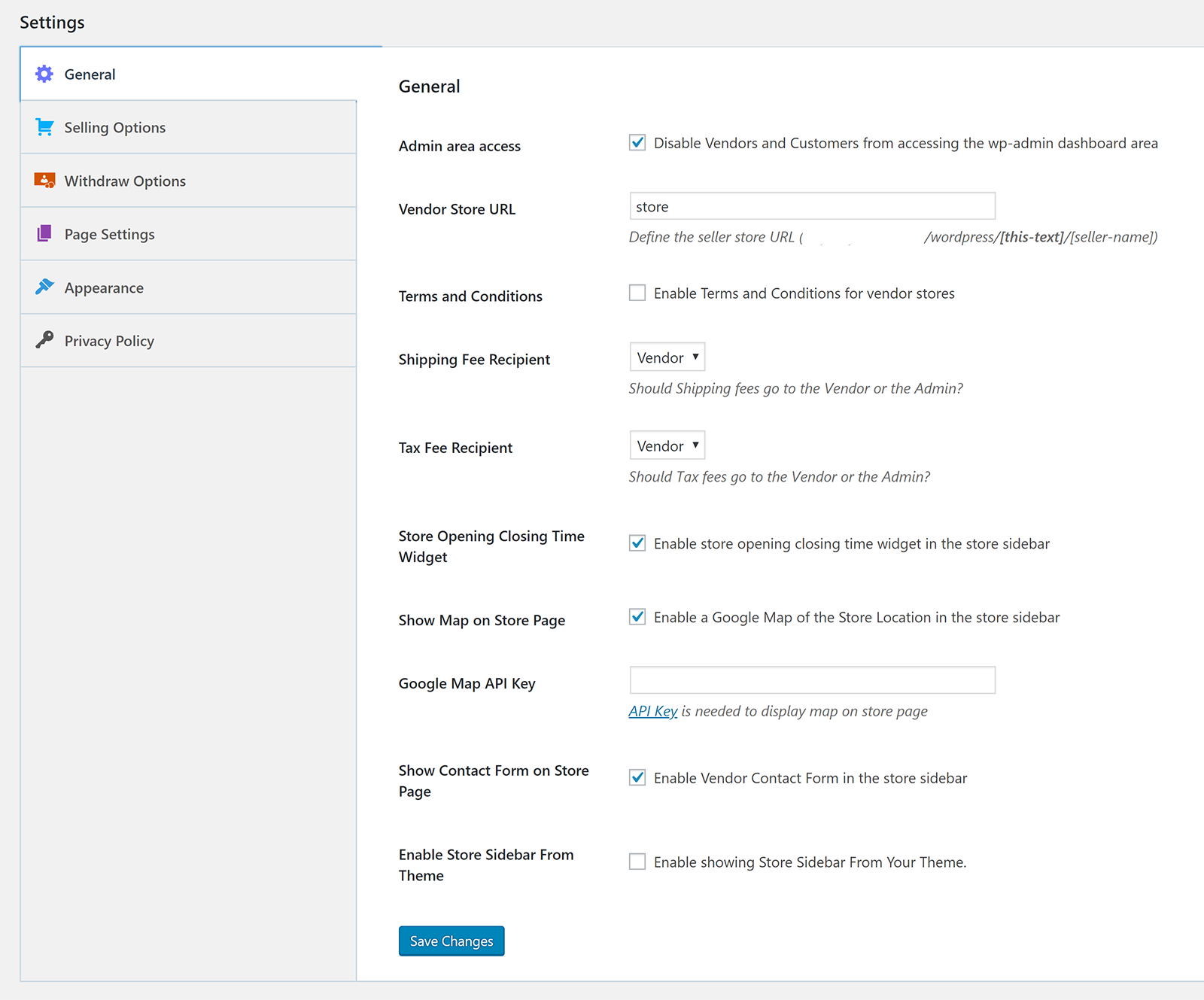The image depicts a settings page with a detailed, structured layout. 

- **Top Section:**
   - The upper left corner of the page features a gray background with the word "Settings" displayed in black text.

- **General Settings:**
   - Below, a white box contains the word "General" in black text accompanied by a blue gear icon to the left.

- **Category Sections:**
   - Under the "General" section, several categories are listed on gray backgrounds:
     - A blue cart icon next to the black text "Selling Options."
     - An orange icon signifies "Withdrawal Options."
     - Two blue pieces of paper beside the text "Settings" in gray.
     - A blue paintbrush next to the word "Appearance" in black.
     - A black key icon with the label "Private Policy."

- **Main Content Area:**
   - The main content area is a white section detailing various settings:
     - "General" is displayed in black.
     - "Admin area access" followed by a blue check mark explaining "Disable vendors and customs from accessing wp-admin dashboard area."
     - "Vendor store URL" displaying "Store, terms and conditions."
     - Sections for "Embedding terms and conditions," "Vendor shipping fee receptor," "Vendor tax fee recipient," and "Vendor store opening and closing time," with a checked box for "Enable store opening and closing widget on the store sidebar."
     - "Show map" in black with a checkmark indicating "Show Google Maps" on the store page.
     - "Google Map API key" field is empty.
     - "Show contact form on store page" enabling vendor contact from the store slider.
     - "Enable store slider from theme," which is unchecked.

- **Bottom Section:**
   - A blue rectangle at the bottom labeled "Save Changes" in white text allows users to save their modifications.